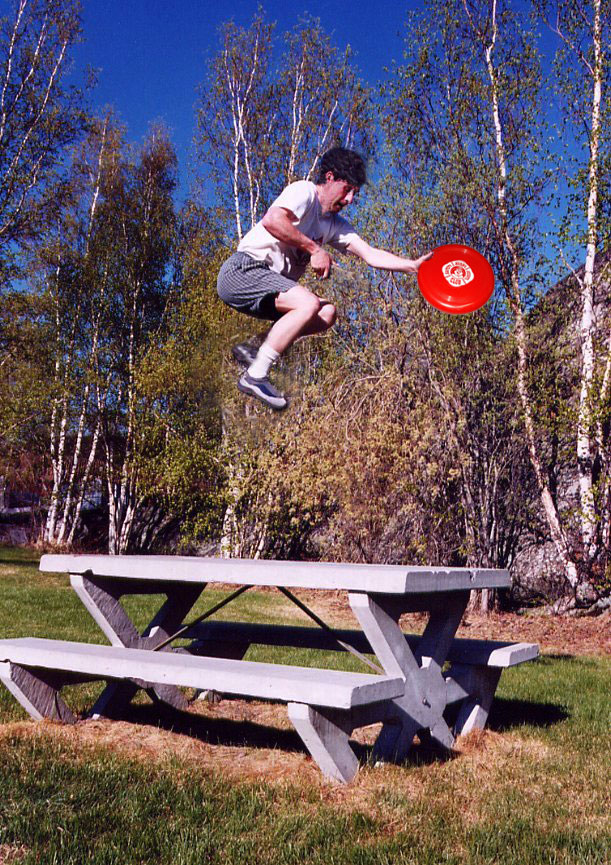The photograph captures a vibrant outdoor scene on what appears to be a warm summer day, characterized by a bright blue sky that forms a striking backdrop. The setting is a park featuring various types of slender trees with whitish bark, possibly aspens or birches, interspersed with some greenery. A white wooden bench with dual seating sides and a tabletop occupies the green and brown grassy area in the foreground. Above this bench, a man is captured mid-air, approximately two to three feet off the ground, seemingly in the middle of an energetic leap. 

He's dressed in a white t-shirt, striped shorts, white socks, and tennis shoes, and he clutches a large red frisbee in his left hand. His short stature relative to the frisbee, combined with an uncanny facial appearance—marked by unusual eyes and a gash-like mouth—imparts a slightly surreal or possibly even AI-generated look to him. His knees are bent, suggesting he's either in the act of catching or simply playing with the frisbee while jumping. Everything about this photo, from the detailed greenery and sparseness of the leaves on the surrounding trees, to the fine distinctions in his attire and the texture of the wooden bench, enhances the lively and slightly peculiar atmosphere of the moment.